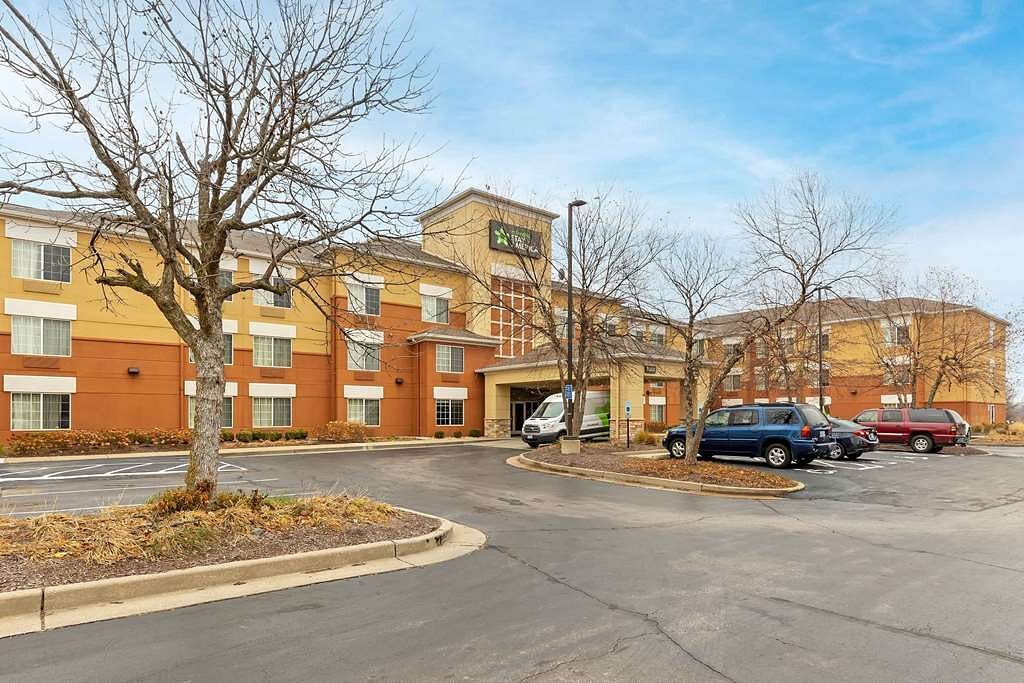The image depicts the entrance of an Extended Stay America hotel, identified by a black sign with a green star at the top. The three-story building features a striking color scheme, with the bottom half painted in burnt orange and the top half in mustard yellow. The facade showcases a tower above the entry doors, extending slightly higher than the three stories, displaying the hotel sign prominently. A driveway leads to a covered greeting area where a white and green hotel shuttle van is parked, suggesting proximity to an airport. The parking lot in the foreground, which has several empty spaces, accommodates three cars: a blue SUV, a gray sedan, and a red SUV truck. Winter is evident in the scene, as the trees are mostly bare of leaves. One tree stands prominently to the left of the image, while several others are scattered in the background under a clear blue sky with wispy clouds. Another wing of the hotel, matching in colors and window patterns, is visible to the right.